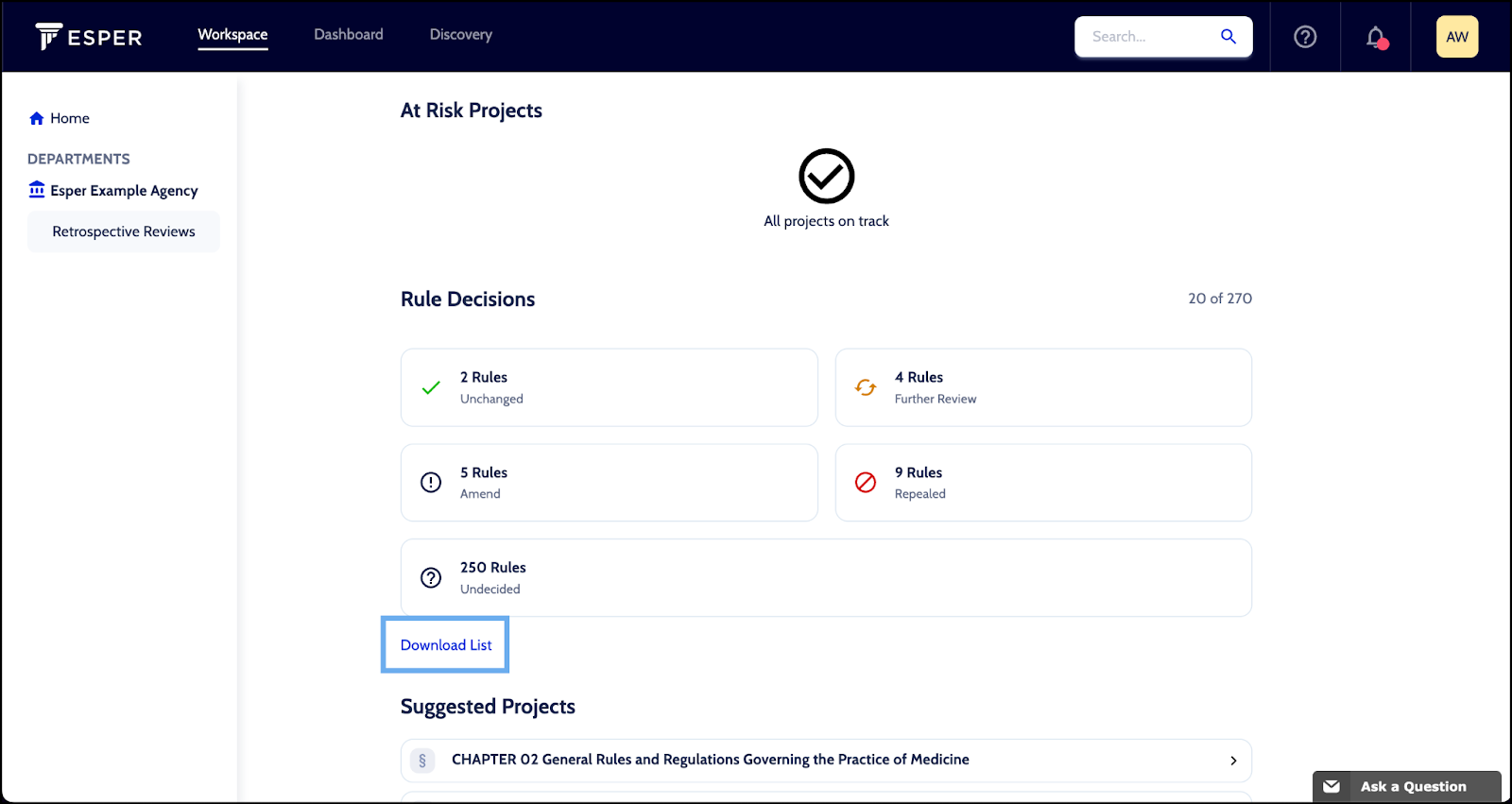The image depicts a web page interface of a platform called Esper. In the top left corner, the Esper logo is displayed on a black navigation bar. The navigation bar contains three tabs: Workspace, Dashboard, and Discovery, with the Workspace tab currently highlighted. On the left side of the page, there is a sidebar menu featuring the Home button followed by a section labeled Departments. Listed under Departments is a specific department named "Esper Example Agency Retrospective Reviews."

The main section of the page, to the right of the sidebar, is titled "At-Risk Projects." A message within this section states that "All Projects are on Track," accompanied by a checkmark. Below this, there is a section named "Rule Decisions," which includes a positive green checkmark next to "2 rules unchanged." Additional categories of 4 rules, 5 rules, 9 rules, and 250 rules are listed but are not checked. At the bottom of the Rule Decisions section, there is a blue box enclosing a link that reads "Download List."